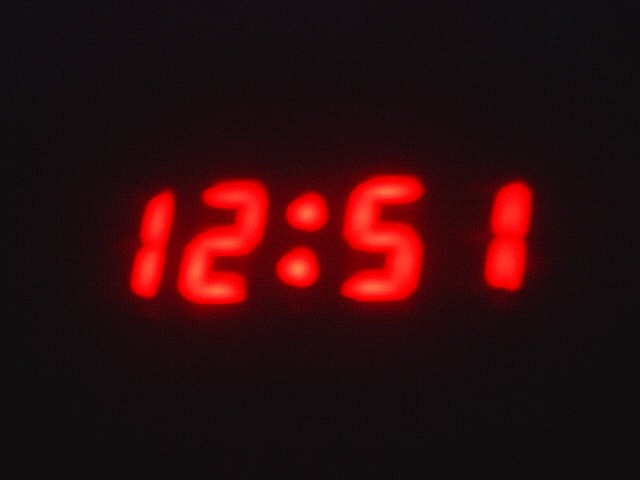This image features a digital clock displaying the time 12:51. The digits are illuminated in vibrant red: a red '1', a red '2', a pair of red dots indicating the separation between hours and minutes, followed by a red '5' and another red '1'. The backdrop is a solid black, providing a stark contrast that makes the red digits stand out prominently. Notably, there is a subtle yellow outline visible within the red segments of the numbers, particularly pronounced in the digits '2' and '5', and distinctly in the small yellow dots at the center of the red dots. This yellow hue is also faintly present in the first '1', though it is less noticeable in the final '1'.